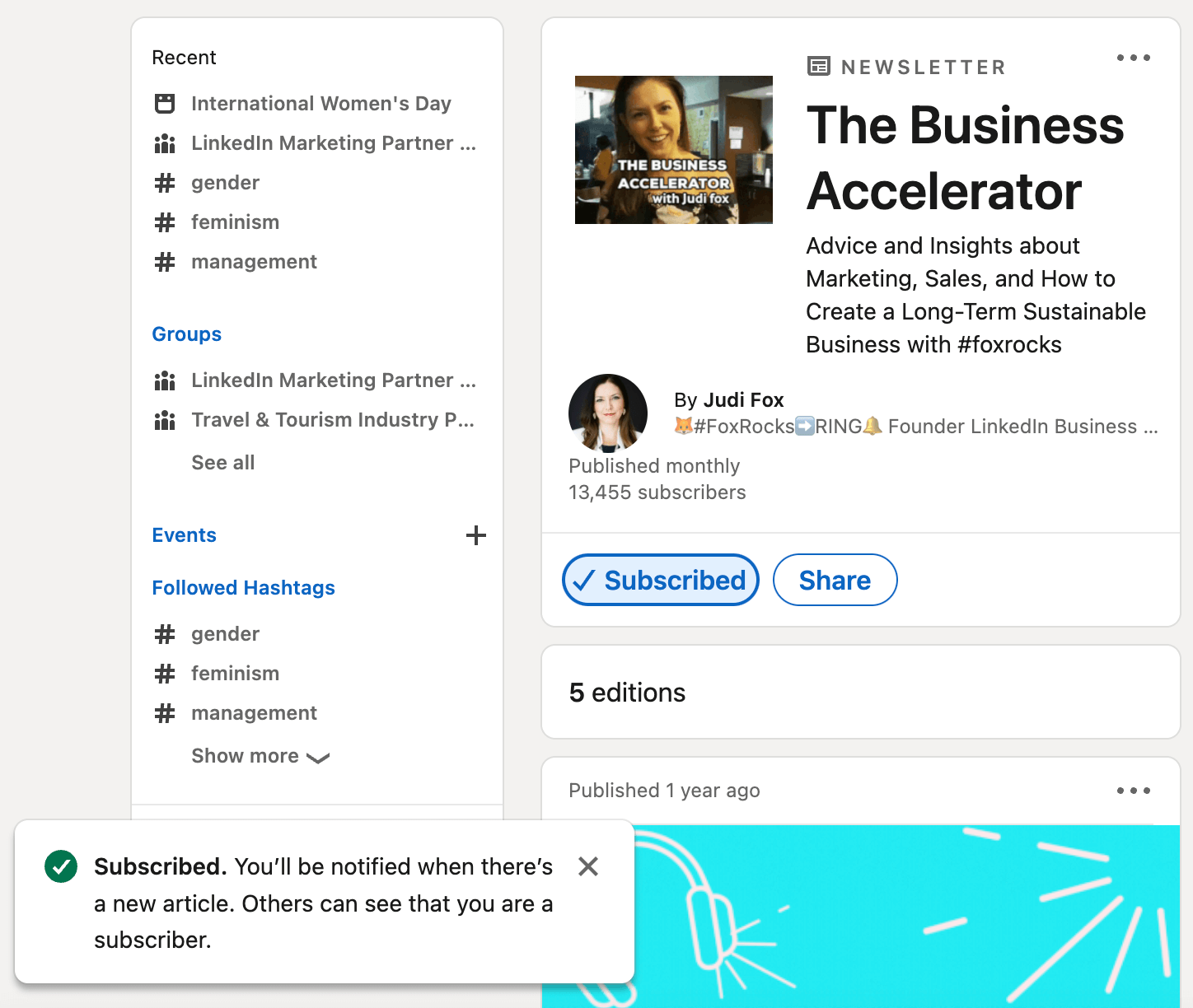### Newsletter: The Business Accelerator

The image displays a detailed layout of a newsletter with a subtle gray background. Prominent white boxes containing various pieces of information are visually striking against the backdrop. 

#### Left-Hand Sidebar:
- **Sections:**
  - **Recent Searches:**
    - "Recent"
    - "International Women's Day"
    - "LinkedIn Marketing Partner"
    - Hashtags:
      - #gender
      - #feminism
      - #management
  - **Groups:**
    - "LinkedIn Marketing Partner"
    - "Travel and Tourism Industry P"
    - [See All]
  - **Events:**
    - Highlighted in blue
  - **Followed Hashtags:**
    - #gender
    - #feminism
    - #management
    - [Show More]

- **Subscription Information:**
  - "You will be notified when a new article is published. Others can see that you are a subscriber."

#### Top Right Corner:
- **Newsletter Title:**
  - "The Business Accelerator" 
  - Provides "advice and insights about marketing, sales, and how to create a long-term sustainable business."
  - Authored by Judy Fox, founder of Fox Racks.
- **Publishing Details:**
  - Published monthly
  - Number of subscribers: 13,455
  - Subscription status indicated by a blue circle around "Subscribed"
  - Sharing option indicated by a white circle around "Share"
  - Five editions published, with the first released one year ago.

#### Image Section:
- **Visual Representation:**
  - Features an image of Judy Fox
  - Accompanied by text: "The Business Accelerator with Judy Fox"

This detailed caption not only organizes but also amplifies the elements within the image, providing clear and comprehensive information for readers.